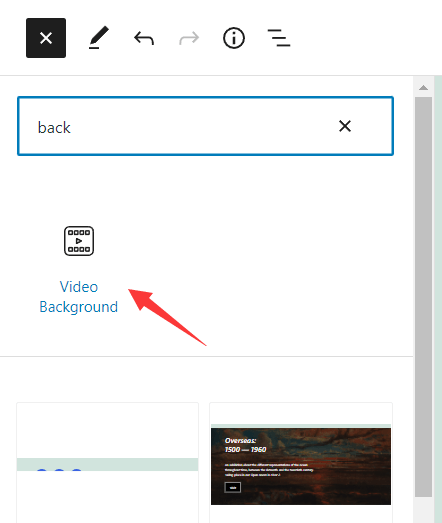The image appears to be a screenshot of a user interface, likely from a software application. 

At the top edge of the image, starting from the left, there are various icons: a white box, a black square, a black pencil with an underline, a black back arrow, a gray forward arrow, a black eye within a circle, and a three-line menu icon suggesting a dropdown menu. Below these icons is a horizontal gray line.

Beneath the gray line, there is a white data field with the word "Back" written inside and outlined in blue. The data field has a black "X" on its right side, indicating a close or delete function. Below the data field, the text "Video background" appears in blue, accompanied by a small video icon above it. A prominent red arrow, seemingly added with a photo editor, points towards this "Video background" text.

Further down, there is another horizontal gray line, followed by two side-by-side rectangular boxes outlined in gray with white interiors. The box on the left has its contents cut off, while the box on the right contains somewhat legible text reading "OVERS," followed by a blurred, possibly "O-E-S," and the numbers "1500 through 1960." The remainder of the text in the right box is too blurred to discern.

The entire interface is set against a background that features blue, red, and gold colors, though the exact nature of the background remains unclear.